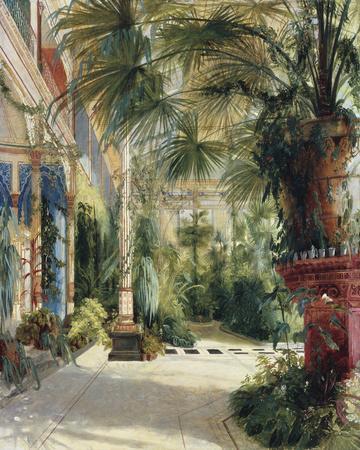An intricate watercolor painting captures a bustling courtyard scene, framed by the weathered facades of buildings and shopfronts on the left and in the background. The ground, paved with cement tiles and dark stepping stones, leads the eye through an organized yet lush environment filled with diverse vegetation. Dominating the scene, numerous palm trees extend gracefully, partially obscuring the structures and merging into the center of the image. Their verdant fronds are echoed by the large, decorative brown pot on the right, which holds the tallest palm and is surrounded by thriving shrubbery. Amidst this verdant growth, clay pots with palm branches are scattered, some precariously stacked, adding to the sense of congestion and natural abundance. The color palette of the painting is vibrant, featuring shades of green, tan, white, blue, orange, and red, highlighting the lively outdoor atmosphere. A striking element is the tall red-brick statue or column adorned with candles, hinting at a historic or cultural significance. The overall effect is a dense and richly detailed portrayal of a garden within an ancient Egyptian-like architectural setting.